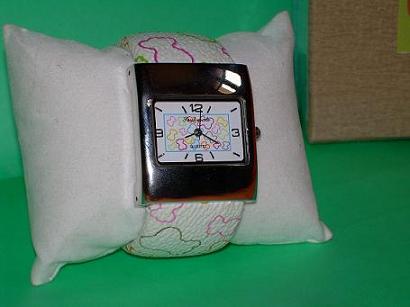This indoor daytime photo features a wristwatch displayed on a small, fluffy white pillow. The watch band is white, adorned with colorful outlines of dog bones, drumsticks, and fish in pastel shades of purple, yellow, blue, and orange. The watch face is a black square with a smaller rectangle inside, containing more of the same colorful images. Time is displayed with thin hour, minute, and second hands indicating 7:20. Only the numbers 12, 3, 6, and 9 are marked, with lines representing the other hours. The setting includes a green background on a hard surface and a partial view of a brown box in the upper left corner.